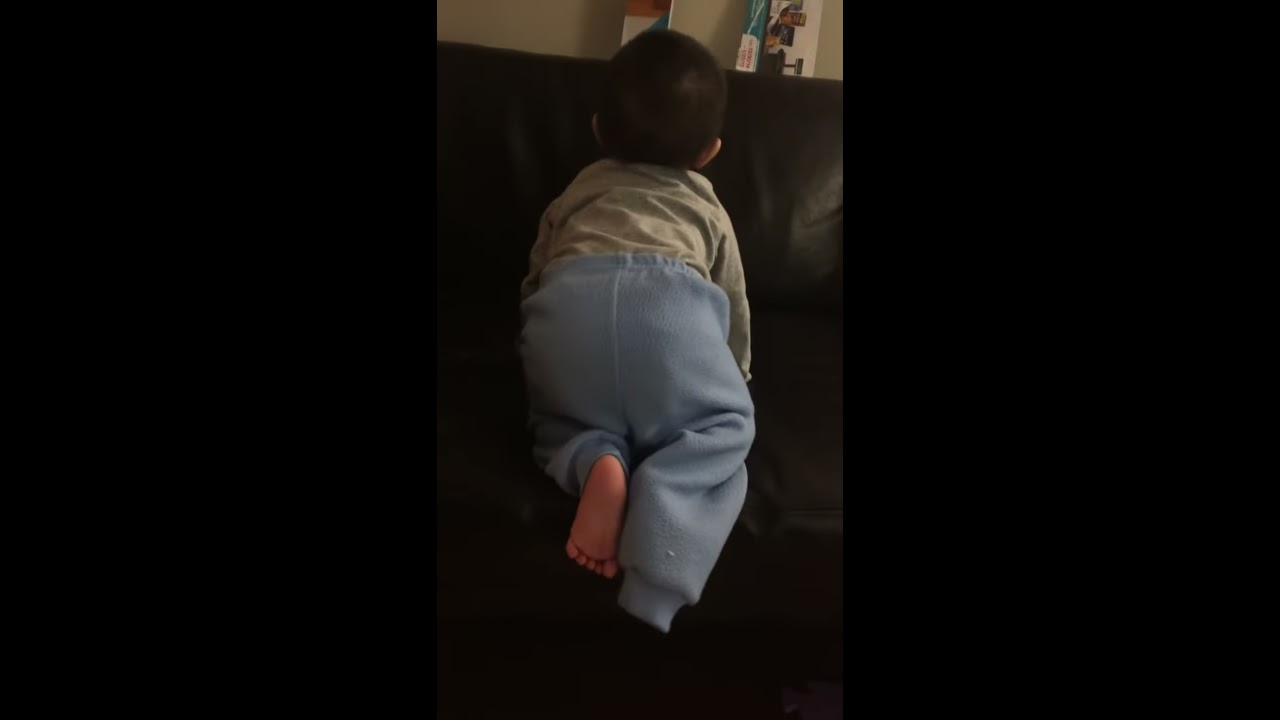In the photograph, a baby with short black hair and dark brown eyes is crawling away from the camera on a black leather couch. The baby is dressed in a long-sleeved gray sweatshirt and powder blue sweatpants, with one foot visible and the other covered by the pants leg. The only exposed foot is pink and bare. The scene is dark with a black background, partially illuminated to show a small portion of a white wall behind the couch. Additionally, there appears to be a toy in the distant background, though it is indistinct. The image is presented within a thick black frame, making the actual photograph approximately 2 inches by 3 inches in size.